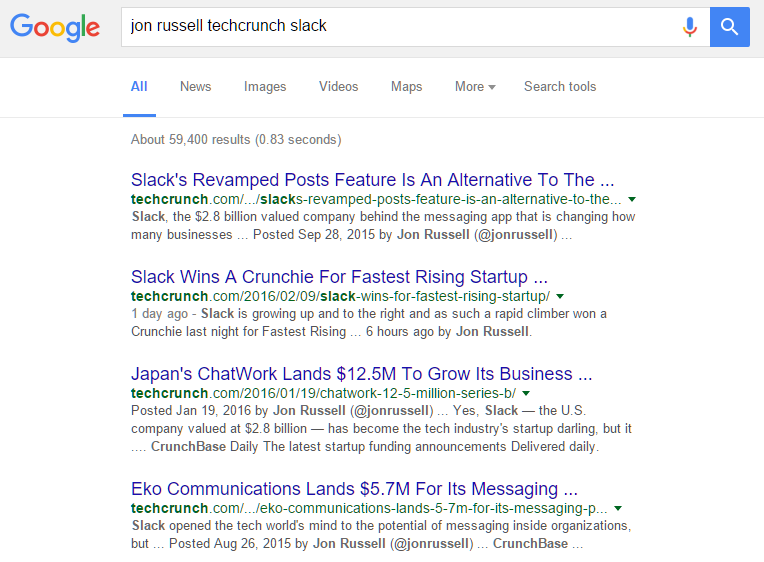In this image, we are looking at a computer screenshot of a Google search results page. The header is light gray, with the Google logo positioned in the upper left corner. To the right of the logo, there is a search bar containing the query "John Russell Tech Crunch Slack" in black text. Flanking the search bar on the right are the Google microphone icon and a blue square with a white magnifying glass.

Directly below the search bar, there is a navigation menu with the options: "All," "News," "Images," "Videos," "Maps," "More," and a pull-down menu, along with "Search tools." The "All" tab is underlined in blue, indicating it is currently selected.

The first search result headline reads, "Slack's revamped post feature is an alternative to," followed by a snippet mentioning "the 2.8 billion valued company behind the messaging app that is changing how many businesses." This result is attributed to John Russell and dated September 28, 2015.

The second search result is titled, "Slack wins a Crunchie for Fastest Rising Startup," and the URL is techcrunch.com/2016/02/09.